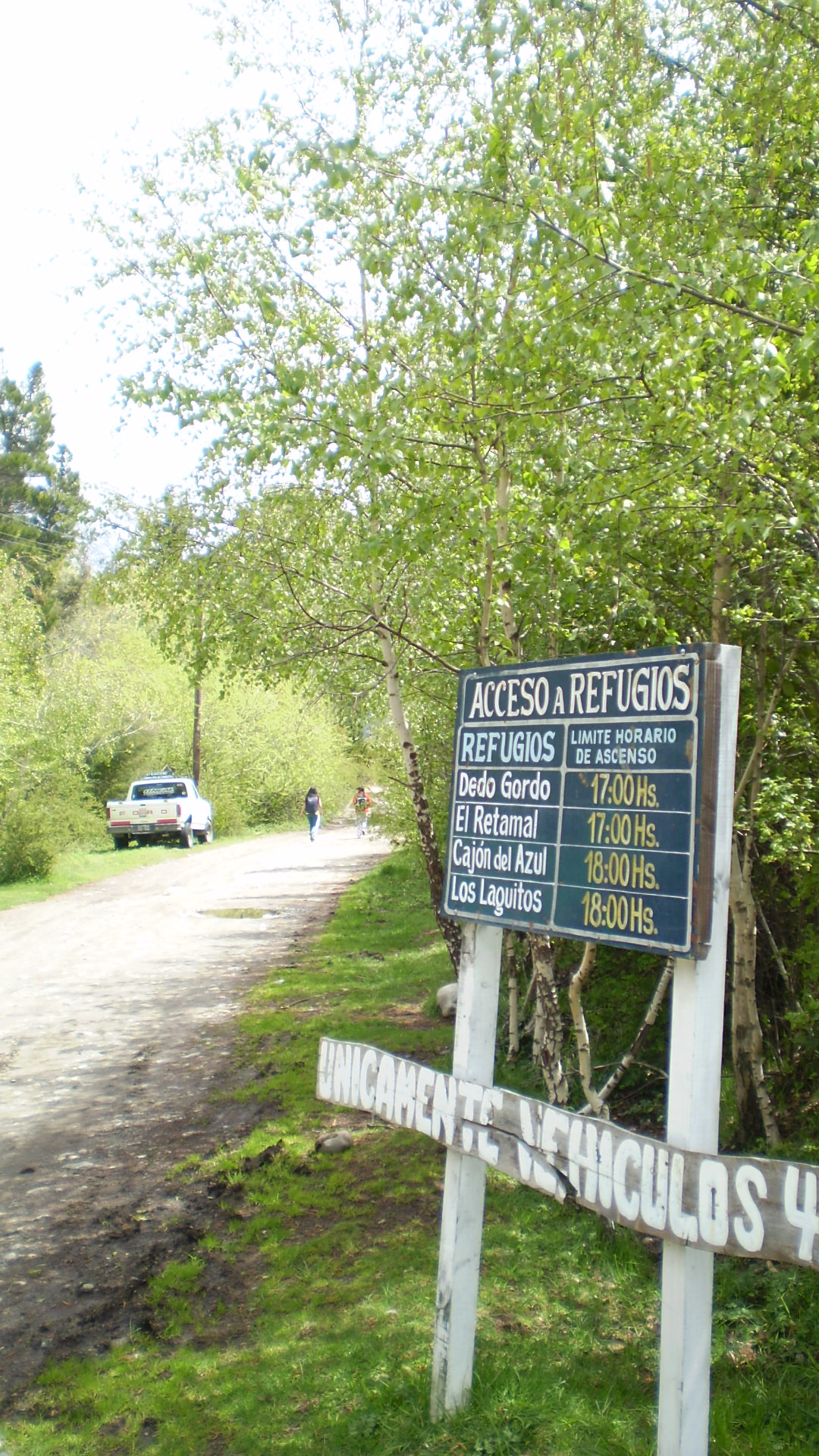The image is a rectangular, color photograph capturing a serene dirt path flanked by lush, green grass and verdant trees. At the beginning of this off-beaten path, situated to the right, stands a wooden sign with white posts adorned with various instructions in Spanish. The sign's blue section prominently reads "ACCESO A REFUGIOS" in white letters, while additional details below, in blue and yellow print, outline further information about access. Adjacent to the path on the left, a white pickup truck is parked on the grass beside a brown telephone pole. Down the center of the dirt road, which is strewn with rocks, two figures with backpacks walk into the distance, bathed in the sunlight that brightens the entire scene.